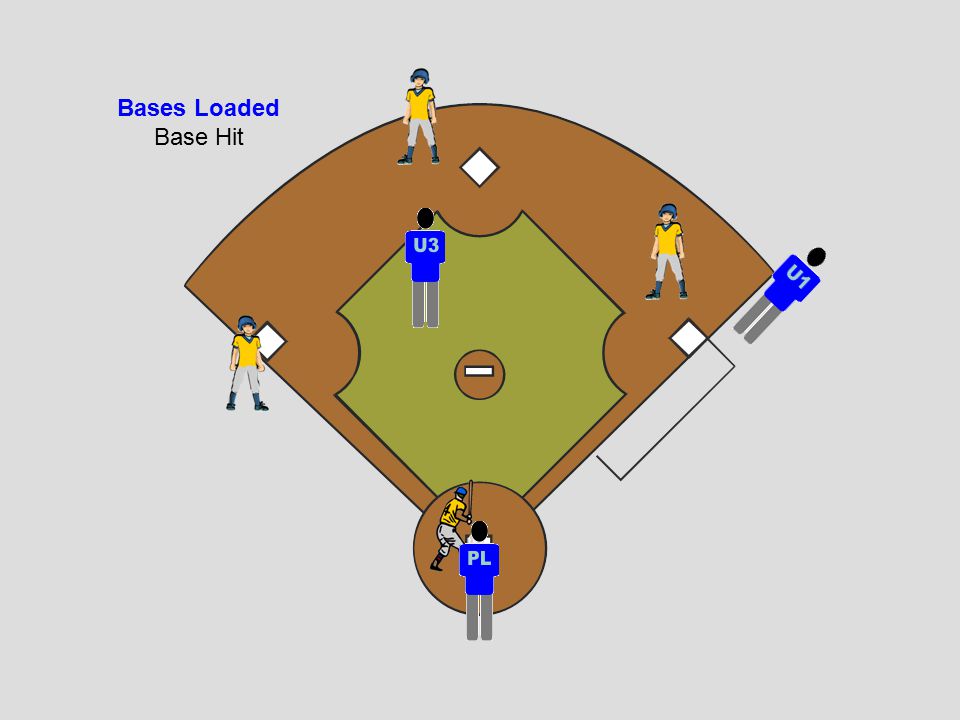The digitally drawn educational image depicts a detailed baseball diamond scenario with two teams. The title "Bases Loaded" is prominently displayed in dark blue letters at the top left, followed by the phrase "Base Hit" in black letters below it. The background features a light grey color, while the infield is depicted with a light brown diamond surrounded by mellow green grass. 

On the diamond, a team in yellow jerseys with blue helmets has runners occupying all three bases, and a batter is positioned at home plate, also in yellow. The opposing team, clad in blue jerseys and gray pants, has players marked with labels indicating their positions: "PL" for the catcher behind home plate, "U1" near first base, and "U3" close to the pitcher's mound. The catcher's figure sports a black head, while the pitching mound is illustrated with a circle and a white line. The image serves as an educational tool, likely to instruct on base-running and fielding scenarios.